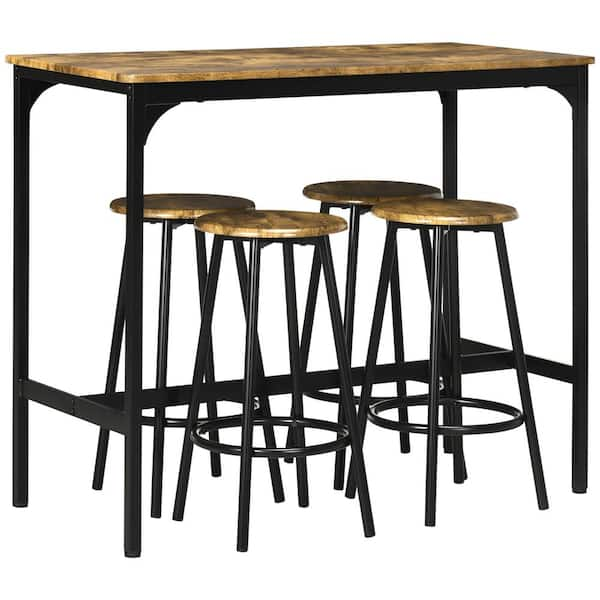The image features a high-top bar table with a wooden surface and black metal legs. The table has four matching bar stools tucked underneath, each with round, copper-colored wooden seats that complement the beige hue of the table's wood. The stools also have black metal legs that fan out slightly at the bottom and are reinforced with a circular black support ring midway down. This sleek and sturdy setup, likely intended for a kitchen, bar, or beer garden, is photographed on a white background, emphasizing its modern and cohesive design.